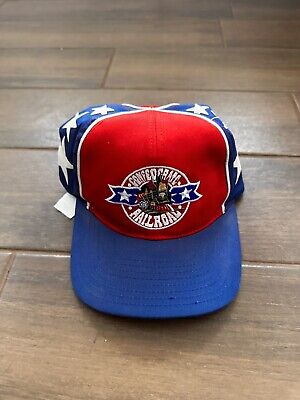This image features a vintage-style baseball cap placed on a brown, grainy, hardwood floor with visible slats. The cap has a striking design: the brim is royal blue, while the front is red. The cap is decorated with white stars set against both colors. At the center of the cap is a circular logo that prominently features the text "Confederate Railroad" in white, encircling an image of a train. Flanking the train image on either side are two stars. Additionally, there is a white tag located on the left side of the cap. The overall look of the cap and the setting evoke a sense of casual, yet detailed, vintage fashion.